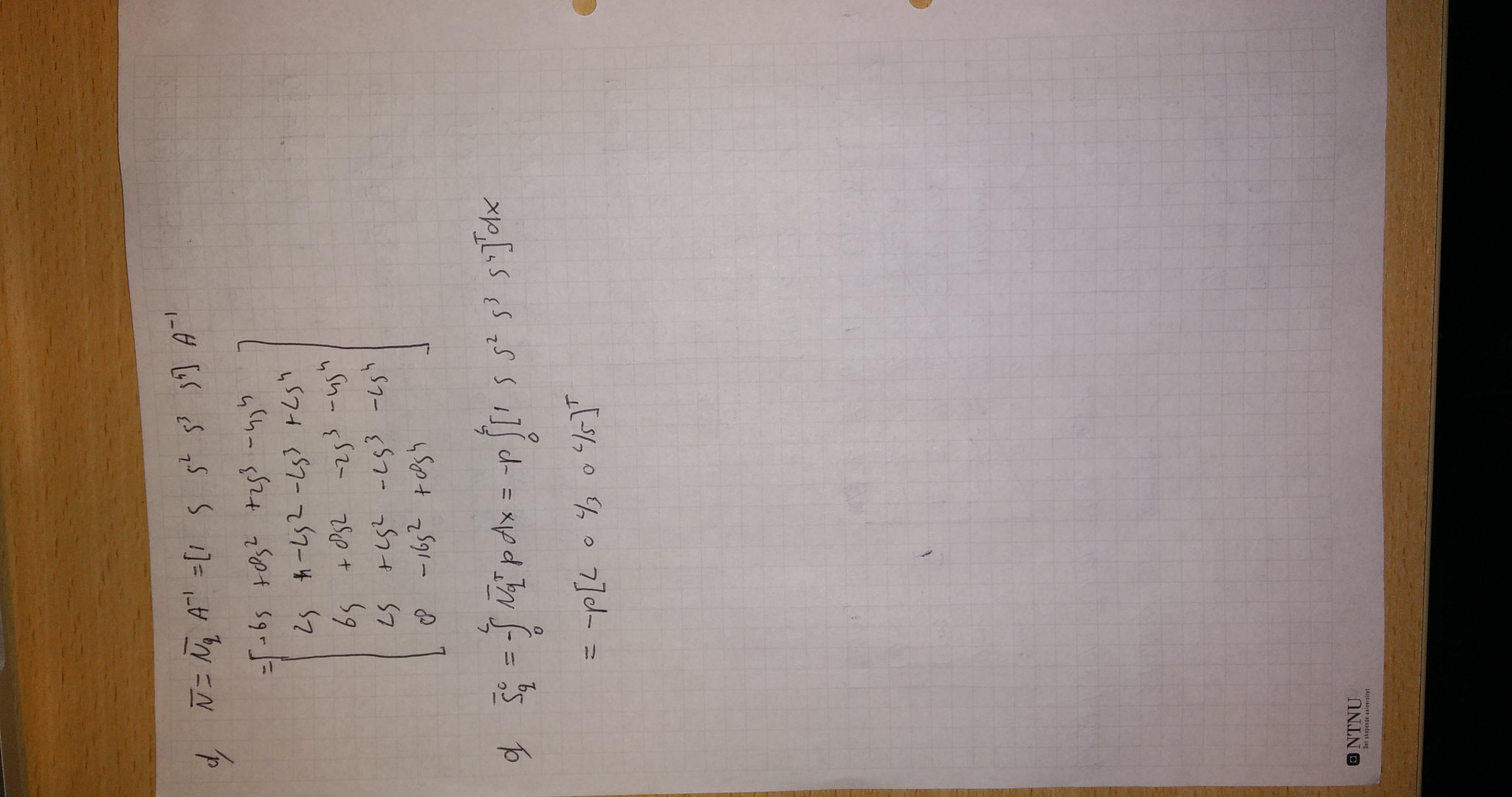The image features a plain white piece of paper, set against a wooden surface that appears to be either a table or a clipboard. This paper is adorned with handwritten equations, primarily involving letters and numbers indicative of algebraic calculations. In the bottom left corner of the paper, the letters "NT" and "U" are prominently visible, suggesting that this may be a college assignment or notes taken by a student. Despite being white, the paper subtly reveals a faint grid pattern, likely from the opposing side, reflected through the paper. Notably, the paper features holes along one edge, indicating it has been torn from a notebook. A small section of the far-right side of the image displays a black background, adding contrast to the composition.